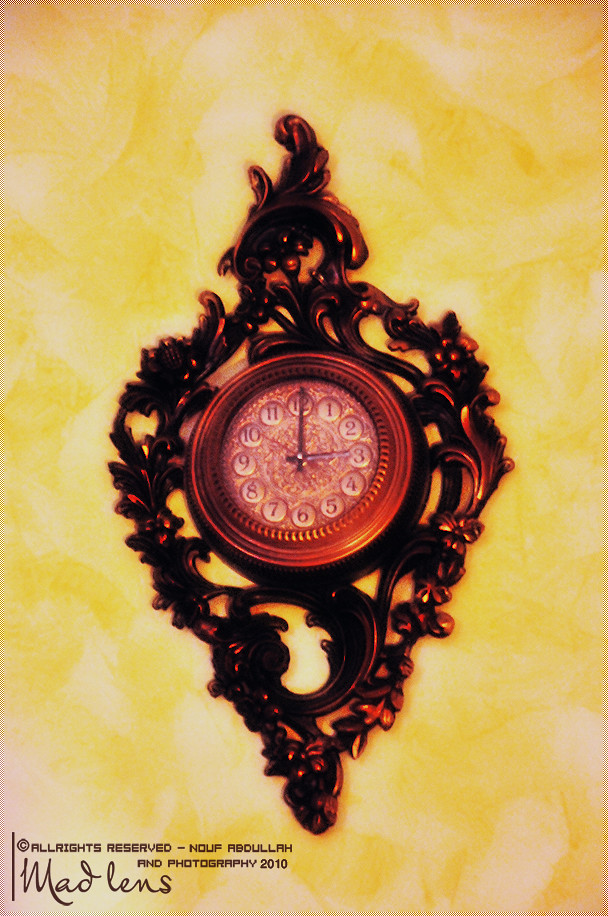This image features an ornate wall clock set against a vivid, almost fiery, yellow and white background that appears to create a burning effect. The clock itself boasts a diamond pattern design with floral motifs, likely crafted from wood or metal, and has a rich, copper-like appearance. The circular center of the clock shares this copper coloring and is embellished with a beaded interior border. The clock face is speckled with shades of white, gold, and red, and features white bubbles enclosing the numbers 1 through 12. The time displayed on the clock is 3 o'clock. In the bottom left corner, there is a copyright notice that reads, "All Rights Reserved, Nowf Abdullah, Photography 2010," followed by the signature "Mad Lens."